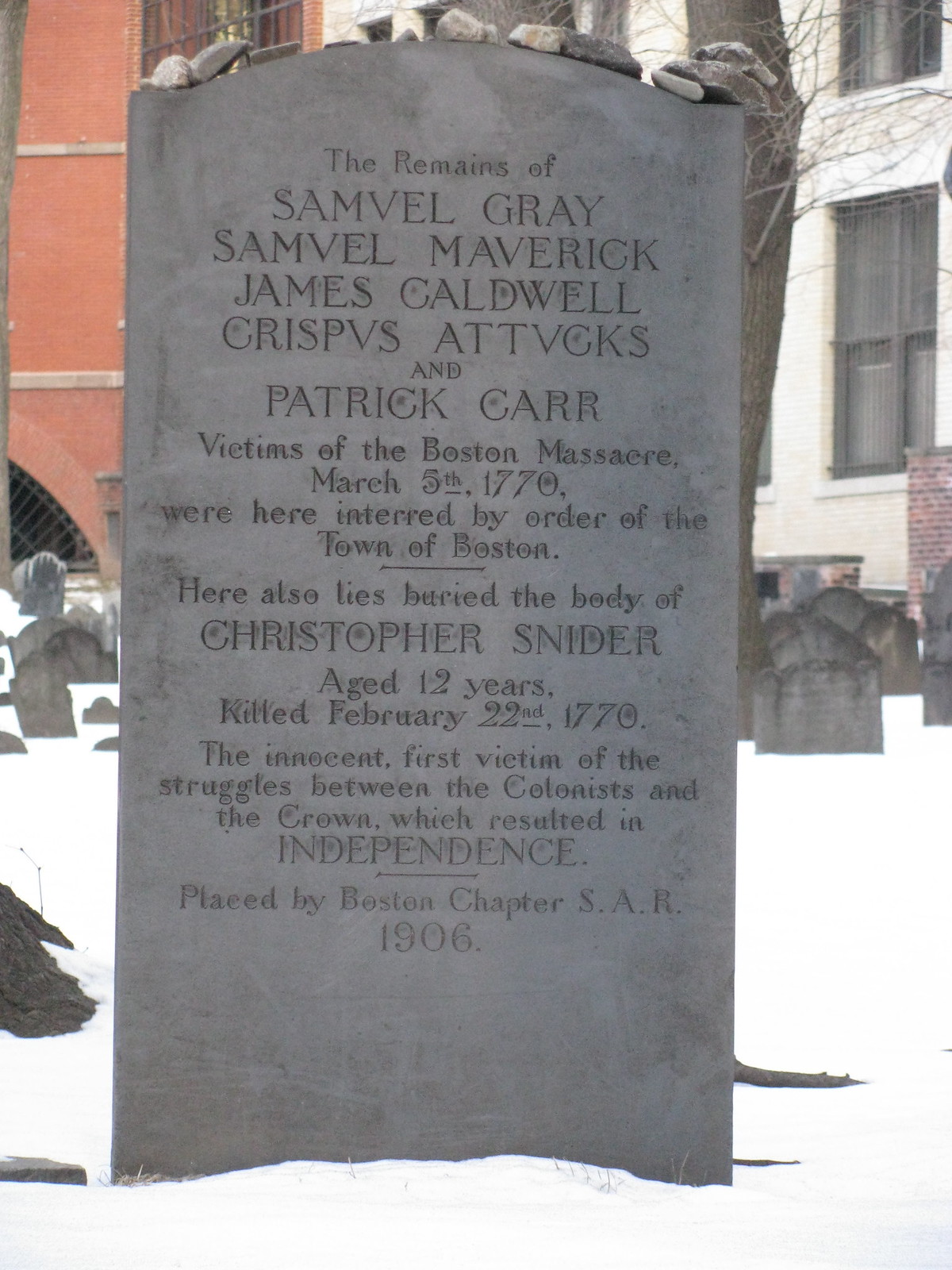In a snow-covered graveyard, set against the backdrop of a red brick building and a tall white structure with windows, stands a prominent gray tombstone. This large, solemn monument is dedicated to the victims of the Boston Massacre, featuring not only the remains of Samuel Gray, Samuel Maverick, James Caldwell, Crispus Attucks, and Patrick Carr, who were killed on March 5th, 1770, but also Christopher Snyder, a 12-year-old boy killed on February 22nd, 1770, recognized as the first innocent victim in the colonial struggle for independence from the crown. The inscription, placed by the Boston Chapter SAR in 1906, commemorates their tragic deaths, with several small rocks left on the stone as tokens of remembrance. Additional tombstones can be seen scattered throughout the graveyard, enhancing the somber and historic atmosphere.